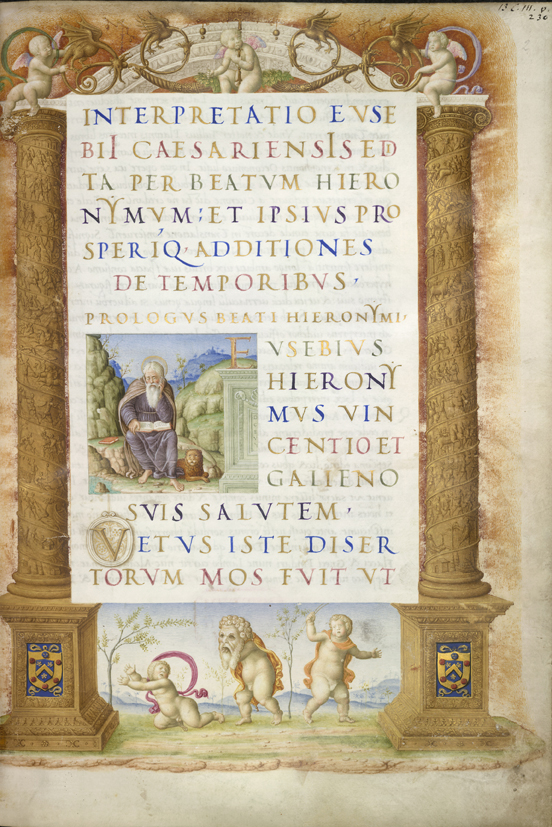The image is a detailed illustration that appears to be a page from a handcrafted, ornate religious text, possibly an old handwritten Bible. The page features intricate artwork and vibrant colors, indicating that it dates back to a time when books were not just written but also considered works of art.

Dominating the image are two elaborate brown columns adorned with a shield at their base. Sitting atop these columns are cherubs or angels, their presence adding to the divine theme of the artwork. Between the columns, a large banner displays text in alternating colors of gold, blue, red, and brown, written in what appears to be Latin. The text is ornate and features phrases like "INTERPRETATIO EVSE" and "BILCAESARIENSED," with other colorful letters spread throughout the page.

At the center, below the text, is a square-shaped painting of a man in a long brown robe and cape, likely from biblical times. He is depicted sitting outdoors with hills and greenery in the background, and there is a lion resting at his feet. This scene is beautifully colorful, with detailed rendering of the man and landscape.

Further down the page, beneath the main banner of text, are three more cherubs, each one looking in different directions, enhancing the intricate and lively nature of the illustration. Additionally, in the far upper right-hand corner, the artwork appears to bear the initials of its author or artist, signifying its handcrafted authenticity. This combination of text, ornate borders, and illustrative imagery marks it as a significant piece of religious and artistic heritage.